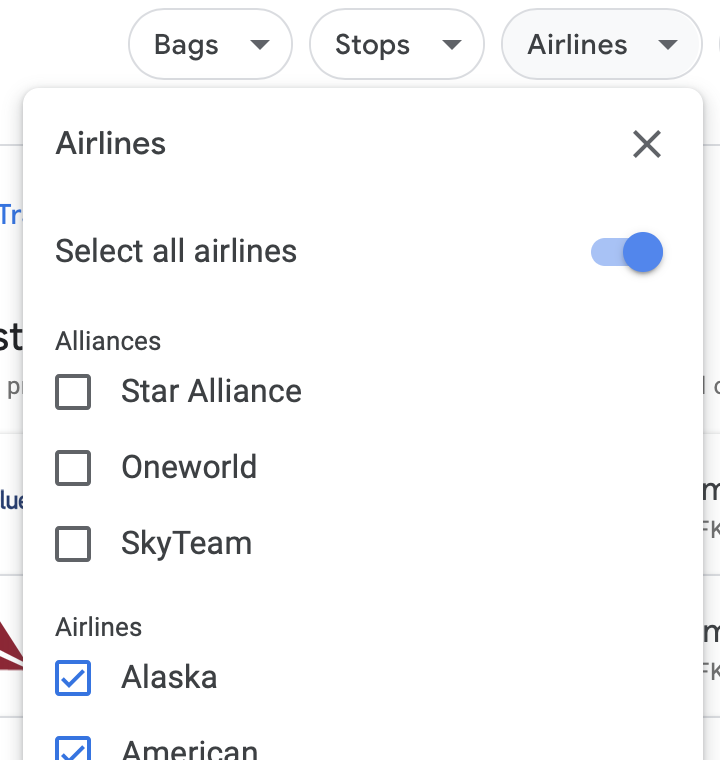The image is a screenshot from an airline website interface with the sides cut off, showing a pop-up box in white text overlaying the main content. At the top of the image, there are three oval-shaped buttons, each outlined with a thin gray line, labeled "Bags," "Stops," and "Airlines" in bold gray font, with drop-down arrows beside each label.

The white pop-up box predominantly displays the "Airlines" section in the upper left-hand corner with an "X" for closing the window in the upper right-hand corner. Just below the title, "Select all airlines" is written, accompanied by a blue toggle slider button positioned to the right, indicating it is activated.

Under the "Select all airlines" section, the word "Alliances" is displayed, followed by three unchecked square boxes labeled "Star Alliance," "OneWorld," and "SkyTeam." Beneath this section, the word "Airlines" is visible, with two checkmarked blue boxes next to the names "Alaska" and "American." The bottom part of the image is cut off, truncating the lower portion of the word "American" and the second checkmarked box.